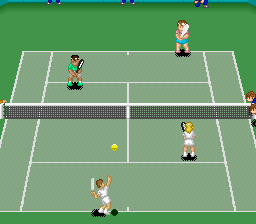This square image captures a retro, overhead view of a vintage tennis video game that dates back to the early days of gaming. The graphics are simplistic, emblematic of the primitive design typical of that era. Central to the scene, a male character with brown hair, dressed in white, is poised in the bottom center, serving the ball which is visibly suspended in mid-air. 

Across the net, positioned towards the right center of the screen, a female player with blonde hair, viewed from behind, stands prepared with her racket in hand, facing the server. In the top left corner of the court, another player, attired in green, is stationed facing the server, ready for the ensuing rally. Finally, in the top right corner, a fourth player, donning a blue skirt and holding a white racket, awaits at the back of the court.

The light green tennis court is framed by a darker green background, with the net stretching horizontally from one side of the image to the other, clearly demarcating the two sides of the court. This charming snapshot from a bygone era of video gaming evokes a sense of nostalgia for simpler times in digital entertainment.